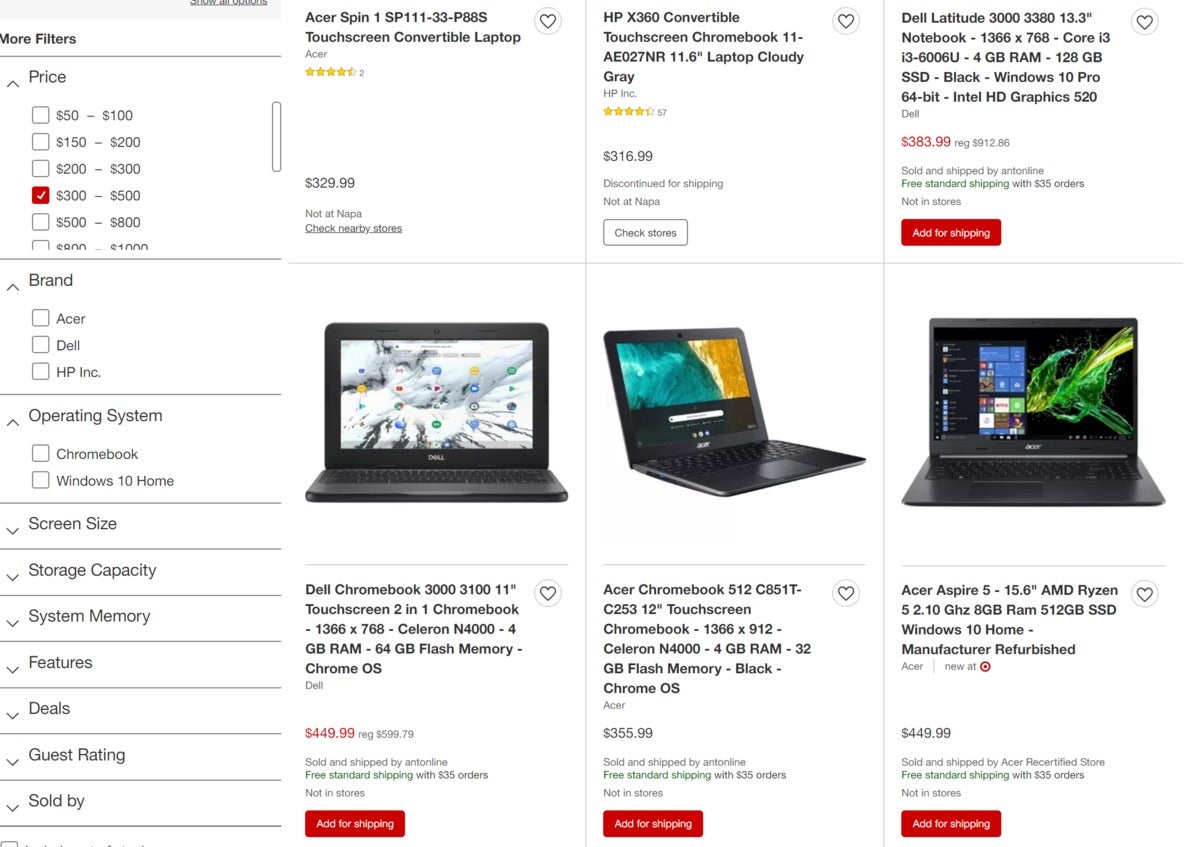The image depicts a screenshot of a technology shopping webpage, specifically for laptops. On the left-hand side, a navigation pane allows users to refine their search with various filters. The first section, "More Filters," includes price categories with checkboxes for different ranges—currently, the $300 to $500 range is selected. Below this, filters for "Brand" are shown displaying options for Acer, Dell, and HP Inc. Further filters for "Operating System" list choices between Chromebook and Windows 10 Home. Additional categories such as Screen Size, Storage Capacity, System Memory, Features, Deals, and Guest Rating are also present, but the complete list is not visible due to the image being cut off.

To the right of the filter column, the main section features a display of six laptop items. Out of these six, only three have accompanying images. The Acer Spin model, listed as a touchscreen convertible laptop, is priced at $329.99 but lacks an image. The HP X360 Convertible Touchscreen Chromebook also has no image but displays its price. Other models listed include the Dell Latitude, Dell Chromebook, Acer Chromebook, and Acer Aspire 5. Below these listings, there are red buttons labeled with phrases like "add for shipping," but the full text is unclear due to the image quality.